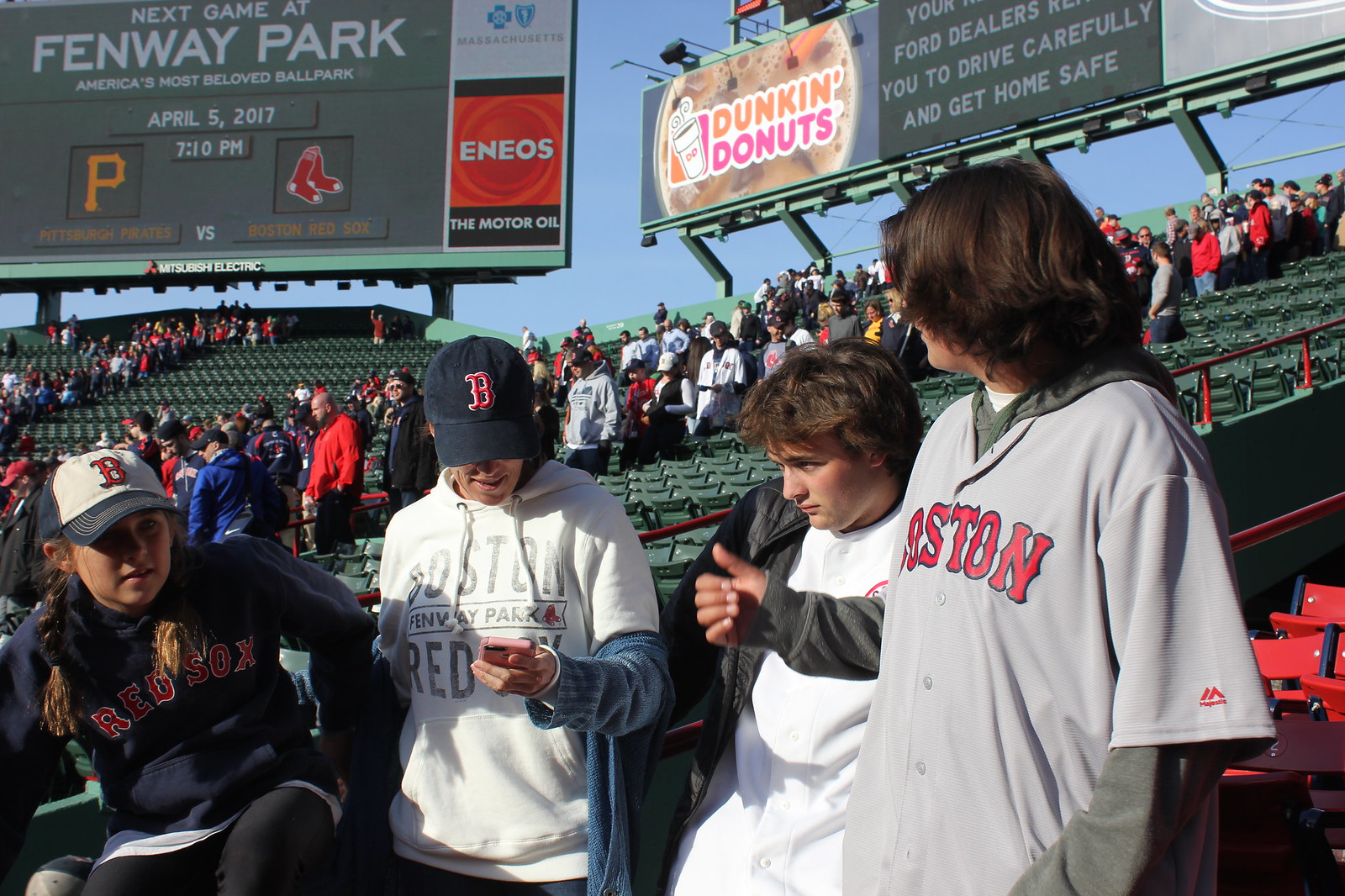This image captures the scene at Fenway Park, renowned as America's most beloved ballpark, where fans are gathering for a baseball game. At the forefront, predominantly centered, are four young fans, all donning Boston Red Sox gear. Starting from the left, a teenage girl with braided blonde hair wears a white baseball cap emblazoned with a red 'B' and a dark blue long-sleeve sweatshirt that has "Red Sox" prominently displayed. She pairs this with blue leggings. To her right is a man sporting a dark blue cap with a red 'B', a white hoodie over a blue shirt, and the word "Red" visible on his attire. Beside him is a young boy, likely around 15, in a white shirt and black jacket looking towards the girl. On the far right, another individual, possibly a woman with shoulder-length dark hair, stands out in an off-white shirt with "Boston" printed across the chest. This person has layered their outfit with an over shirt, red leggings, a green full-sleeve hoodie, and a white t-shirt underneath.

The background reveals several rows of stands filled with a mix of people filing in and vacant seats. Above, numerous billboards are visible. The scoreboard at the top left announces the next game, scheduled for April 5, 2017, at 7:10 PM, featuring the Boston Red Sox against the Pittsburgh Pirates. The scoreboard branding includes Mitsubishi Electric, with logos of Massachusetts and Enios motor oil also in sight. Additional advertisements include Dunkin Donuts and a public safety message encouraging careful driving. The vibrant colors of the image—ranging from gray, red, blue, green, to orange, pink, and purple—add to the lively, anticipatory atmosphere of a sunny day at Fenway Park.